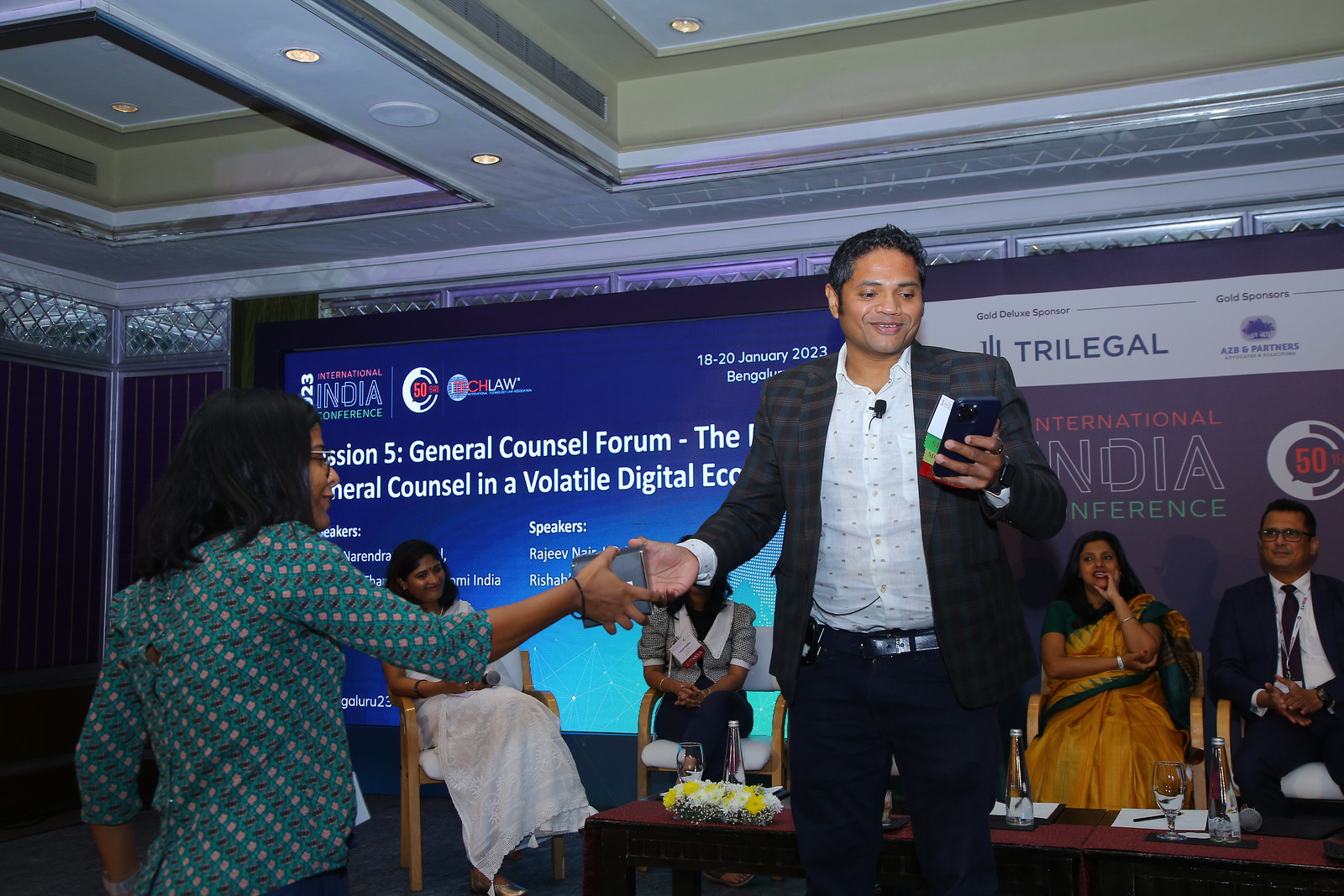The image depicts an opulent ballroom setting, likely in a hotel, featuring intricate crown molding and raised ceilings supported by decorative beams. The scene is set for a professional conference, evident by the blue and purple screens in the background. One screen on the left displays titles such as "Session 5: General Counsel Forum in a Volatile Digital Economy," partially obscured by attendees. Standing prominently in the foreground is a man in a checkered jacket, intently examining something in his left hand while smiling. He seems to be receiving an item, possibly a plaque, from a woman in a green shirt. Behind them, five individuals, a mix of men in suits and a woman in bright yellow Indian attire, are seated at a table on stage. To the right, a large banner adorned with white and purple borders reads "Tri-Legal India Experience," reinforcing the international and Indian context of the event. Additional attendees are visible, either standing or seated in chairs, further emphasizing the formal and engaging atmosphere of the conference.